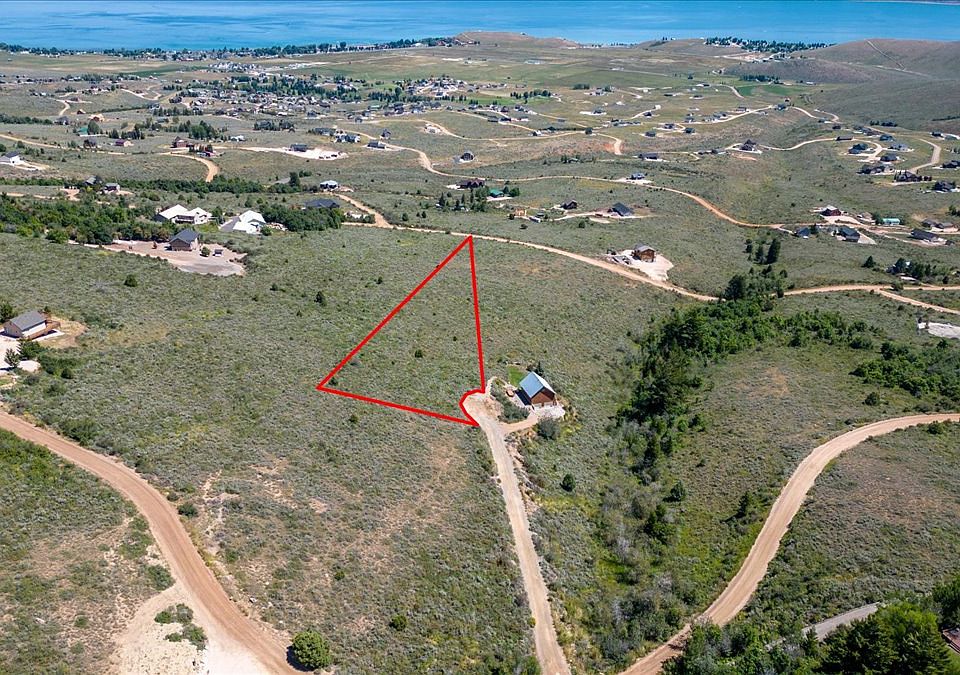This color aerial photograph captures a sprawling rural landscape with a combination of grassland, dirt roads, and scattered houses. In the foreground, the land is green with patches of brown, indicating dry or sparse vegetation. Scattered throughout the landscape are clusters of trees in varying sizes and shapes, with dark green foliage. The terrain is slightly hilly and mostly covered in brush or grass, resembling dry land used for grazing cattle.

In the background, there's a medium blue-toned large body of water with visible waves or choppiness. The shoreline transitions into the lush green mainland. Dirt roads crisscross the entire area, connecting isolated houses and clusters of houses. Towards the top left corner of the image, a small town can be seen, characterized by a denser grouping of buildings.

At the center of the image is a prominent red triangle, seemingly drawn as a marker. The triangle's bottom right corner has a distinctive inward curve that wraps around a dirt driveway near a solitary barn adjacent to one of the isolated houses. This triangular marker stands out in the rural scenery, adding a unique focal point to the overall countryside vista.